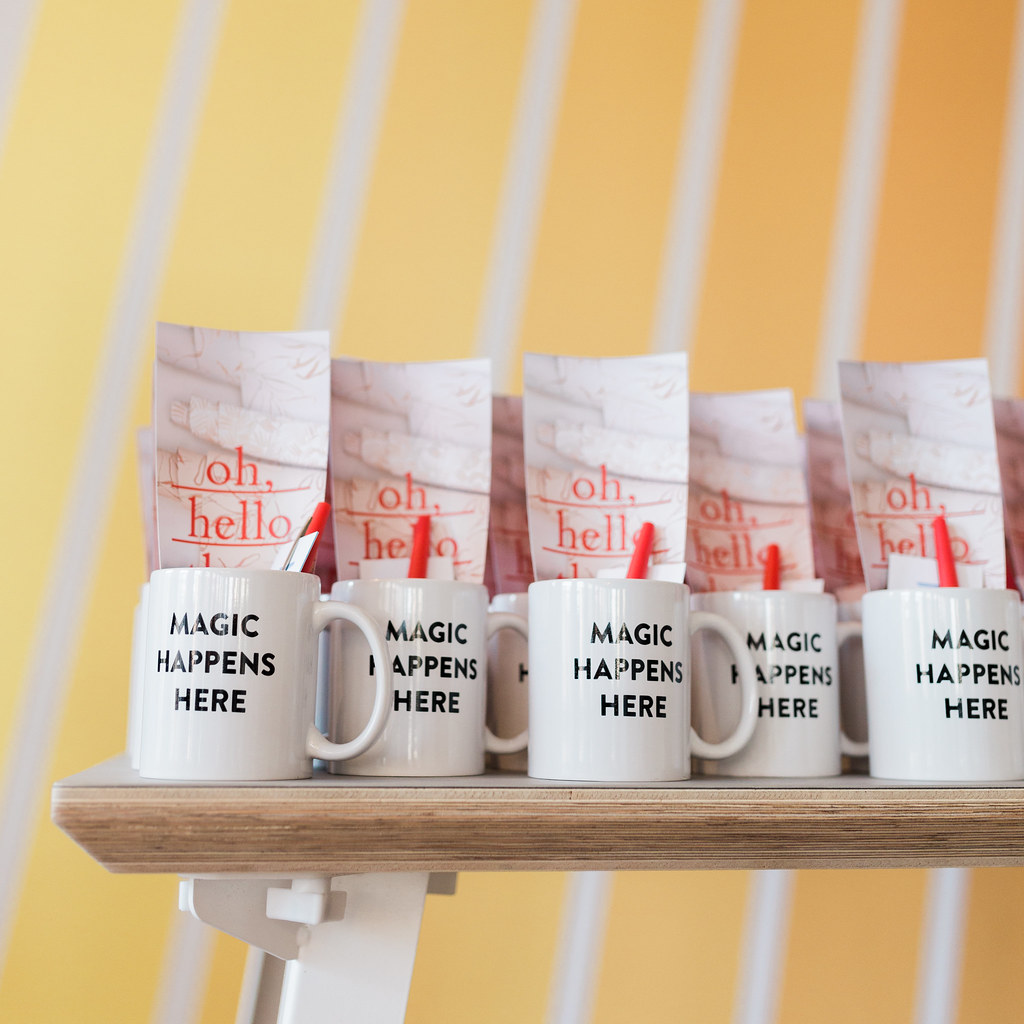The image depicts a wooden brown shelf adorned with five identical white mugs, all lined up neatly in front and backed by a few additional mugs. Each mug bears the inscription "MAGIC HAPPENS HERE" in bold black capital letters. Inside the mugs, there are pieces of rectangular paper, largely obscured but partially visible with the text "OH HELLO" written on them. Some of these papers seem to have an additional, unreadable message extending into the mugs. Additionally, each mug contains a red object that looks either like a pen or a straw, positioned through the paper. The backdrop consists of a yellow surface with thick, slightly diagonal white stripes, adding an eye-catching contrast to the scene.